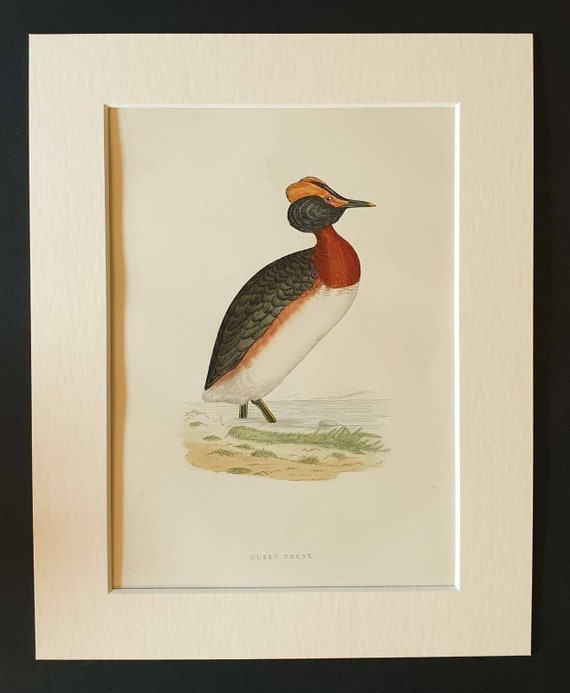This image features a watercolor painting of a bird, specifically a "Dusky Grebe," encased in a black frame with a white matting. The centered painting is slightly indented, creating a distinct separation from the matting. The bird, facing to the right, is depicted standing in light blue water with green and brown sand around its legs. It has a striking appearance: an orange marking on its head, a black beak and head, a burgundy-colored neck and upper chest, a white underbelly, and black feathers on its back. The background of the painting is primarily white, enhancing the bird's vivid colors.